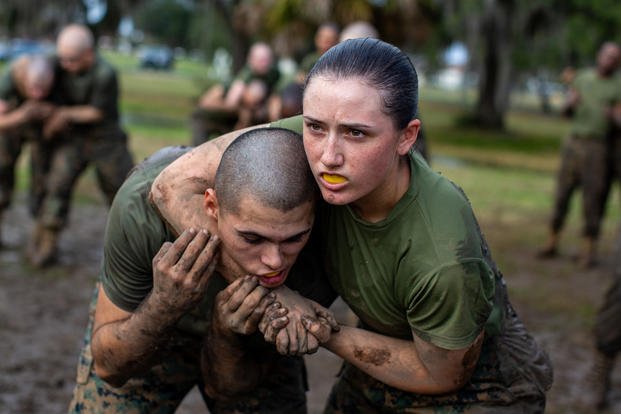This photograph captures a military training exercise, featuring a pair of individuals engaged in combat training amidst a muddy outdoor environment. Centralized in the frame are a man and a woman, both clad in green t-shirts and camouflage pants, which suggest a military uniform. The man, positioned on the left, has short, dark, buzz-cut hair and extremely muddy hands, while he is bent forward. The woman on the right, distinguishable by her dark hair tied back in a ponytail and a yellow teeth guard in her mouth, has him in a firm headlock, her arm wrapped around his neck as he grips her forearm. Despite the intense action, the man does not appear overly distressed, implying a controlled training scenario. Both individuals are heavily muddied, underscoring the rigorous nature of their exercise. The blurred background reveals multiple pairs of other participants similarly engaged in training, surrounded by a muddy field with trees and patches of grass in the distance.